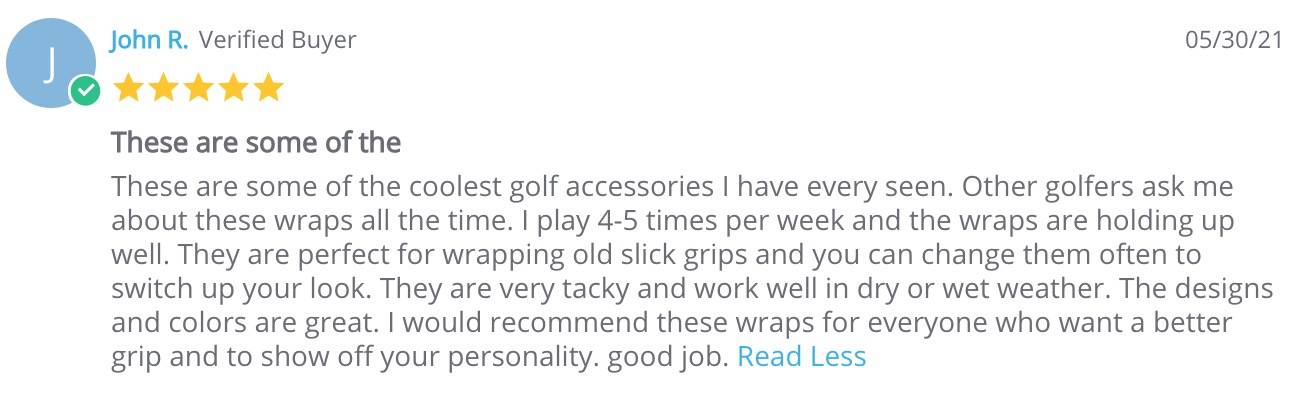"A screenshot of an online review is displayed prominently. At the top left corner, a solid blue circle contains the initial 'J,' signifying the reviewer's profile icon. To its right, a green circle outlined in white and featuring a white checkmark denotes a verified purchase. The review is authored by 'John R.' and is dated May 30, 2021. Accompanying the name are five gold stars, indicating a perfect rating.

The review itself stands out with the first line in bold black text, 'These are some of the coolest golf accessories I've ever seen.' He goes on to describe how other golfers frequently inquire about his gloves. John reveals that he plays golf four to five times a week and praises the wraps for their durability, noting that they are excellent for rejuvenating old stick grips and can be easily replaced as needed. He highlights their tackiness, mentioning their effectiveness in both dry and wet conditions. John is also impressed by the various designs and colors available, recommending these wraps to anyone seeking a better grip and a chance to show off their personality. He concludes with a commendation, 'Good job.'

At the very end, the word 'relax' is displayed in blue text, providing a serene closure to the review."